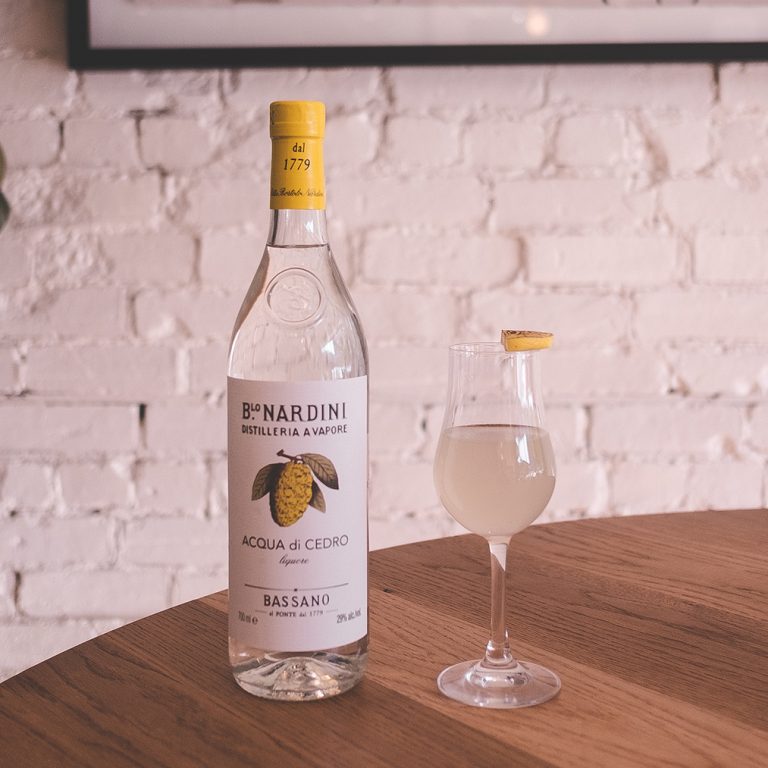In the photograph, a clear glass bottle and a stemmed glass goblet sit on a round wooden table with a pronounced woodgrain texture. The bottle, featuring a distinctive yellow lid inscribed with "Dahl 1779," boasts a white label adorned with an illustration of a yellow fruit with green leaves and text that reads "Acqua di Cedro." The label, further detailed with the words "B-L-O Nardini Distilleria di Vapor," also indicates the bottle contains 29% alcohol. To the right of the bottle, the goblet holds a murky white liquid, likely lemonade, topped with a slice of lemon. The setting is inside a room with white-painted brick walls that reveal some rough texture beneath the paint. Above the scene, a large black-framed picture, partially cut off, adds to the decor without revealing its content.